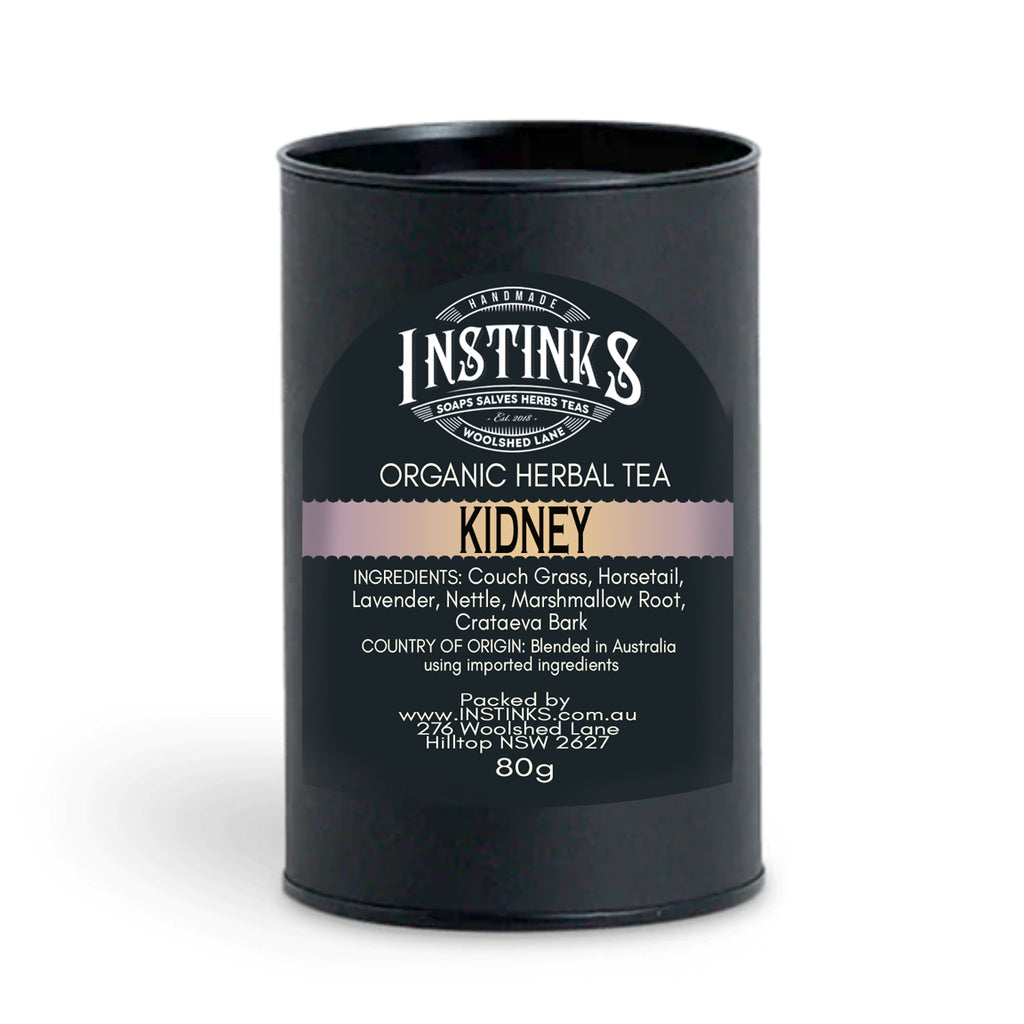The image depicts a black cylindrical container of organic herbal tea against a white background. The container features a blacker central logo labeled “Handmade Instincts Soaps, Salves, Herbs, and Teas” followed by an address, "276 Wool Shed Lane, Hilltop NSW 2627." In gold lettering beneath the logo, it reads "Organic Herbal Tea." Below that, on a contrasting pink strip, the word "Kidney" is printed in black text. The detailed list of ingredients, including couch grass, horsetail, lavender, nettle, marshmallow root, and krataiva bark, is written in white. The label also specifies that the product is blended in Australia using imported ingredients. Packaging information includes the website, www.instincts.com.au, at the bottom of the label.